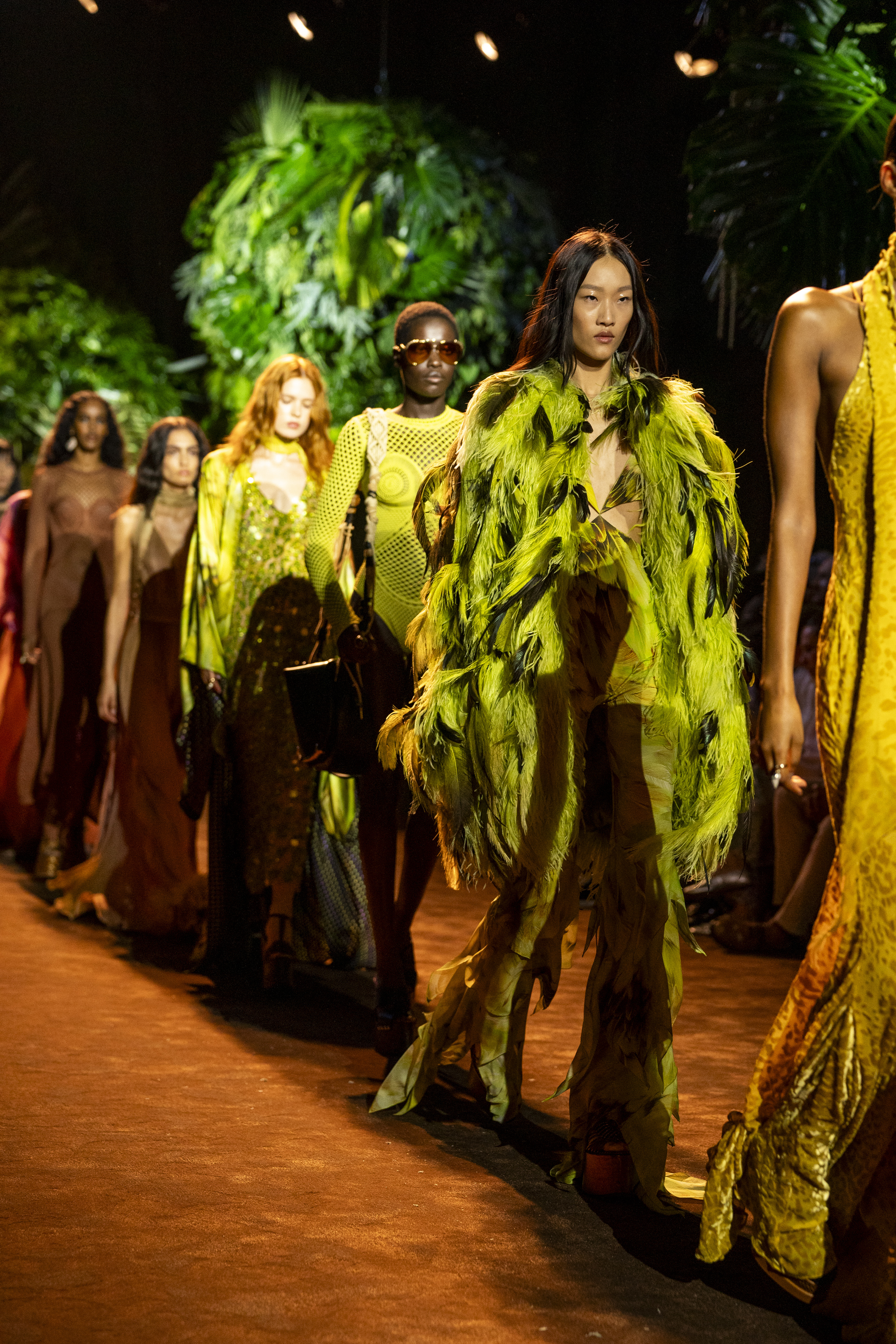In this detailed image of a fashion runway exhibition, six diverse models are showcased in jungle-inspired attires, lined up against a backdrop of circular-shaped, plastic trees and illuminated by studio lights. The runway itself has an orange, rough texture resembling earthy ground. Starting from the front, the first model is partially visible, donning a long, form-fitting gold pantsuit. The second model, an Asian woman, stands out in a green and black feathered jacket paired with loose-fitting pants and high heels, creating a strikingly fluffy appearance. The third model, an African-American woman with closely cropped hair and sunglasses, wears a yellow mesh bodysuit accented with thicker pieces resembling a bikini. Moving further back, the fourth model, a red-haired woman, sports a brown and greenish-yellow outfit with an algae-like texture. The fifth and sixth models are adorned in reptile-scale-like dresses, with the fifth model's dress shimmering and the sixth model's outfit, a brownish skirt, appearing more porous and aerodynamic. Together, their vivid costumes and varied ethnicities create a vibrant, eclectic display on this contemporary, jungle-themed runway.